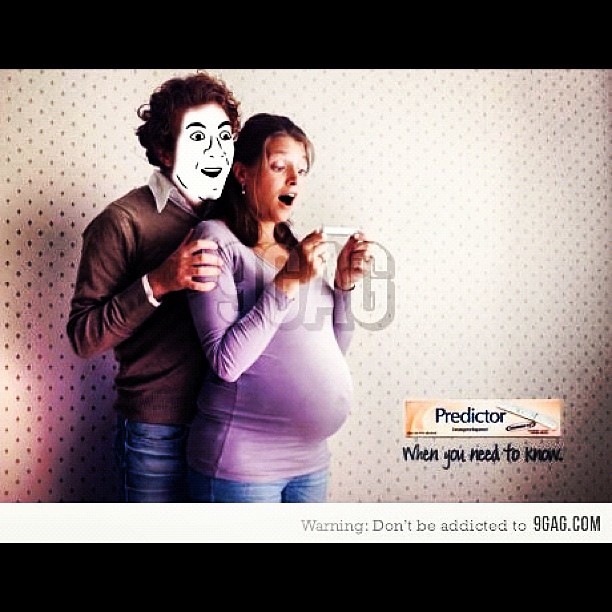In this photograph, framed by black stripes at the top and bottom, a young and visibly pregnant woman, wearing a light purple shirt, stands against a white wall adorned with black polka dots. She is holding a pregnancy test at chest-height with her hands, and her mouth is open in a wide, shocked expression. Behind her, a man dressed in a brown sweater and jeans looks over her shoulder, gently holding onto it. His face, manipulated into a black and white cartoonish "shocked" meme expression, contrasts sharply with the realistic setting. In the bottom right corner of the image, there is an image of a pregnancy test with the label "Predictor" and the slogan "When you need to know." Below this, a warning reads, "Don't be addicted to 9gag.com."